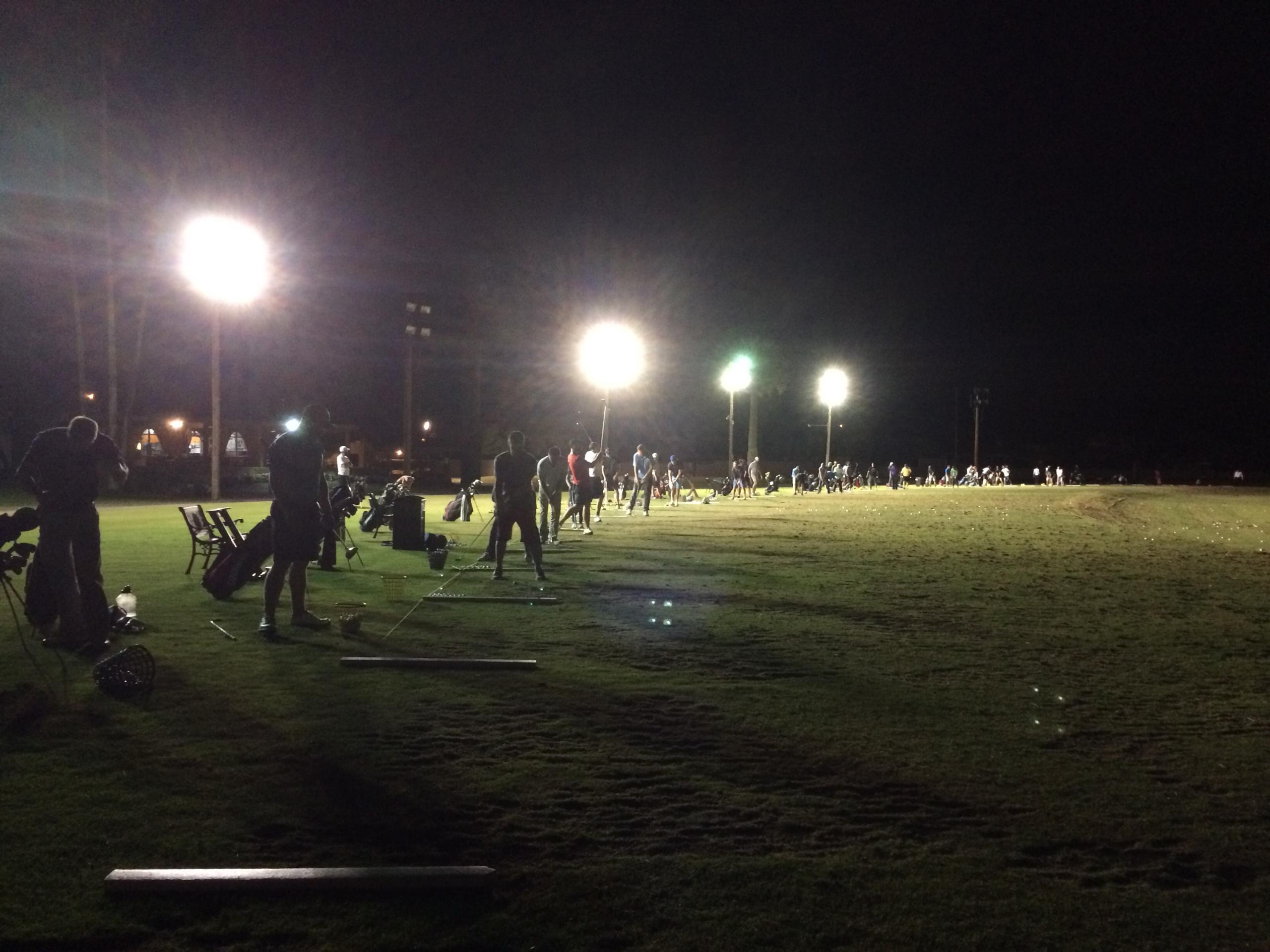This non-professional photo captures a nighttime scene at a golf driving range. The image is quite dark, making it difficult to discern faces, but the bright stadium-style spotlights illuminate a row of golfers on the left side, each poised to take a swing. The field, covered in short, green grass, sprawls out before them. In the background, a clubhouse with lit windows glows softly, offering a hint of warmth and activity. The scene suggests an event, given the number of golfers and the vague silhouettes of a crowd, possibly friends and family, gathered in the distance. Among the indistinct figures, one golfer wearing a red t-shirt stands out, having just completed his swing, while the rest blend into the dark sky as mere silhouettes.